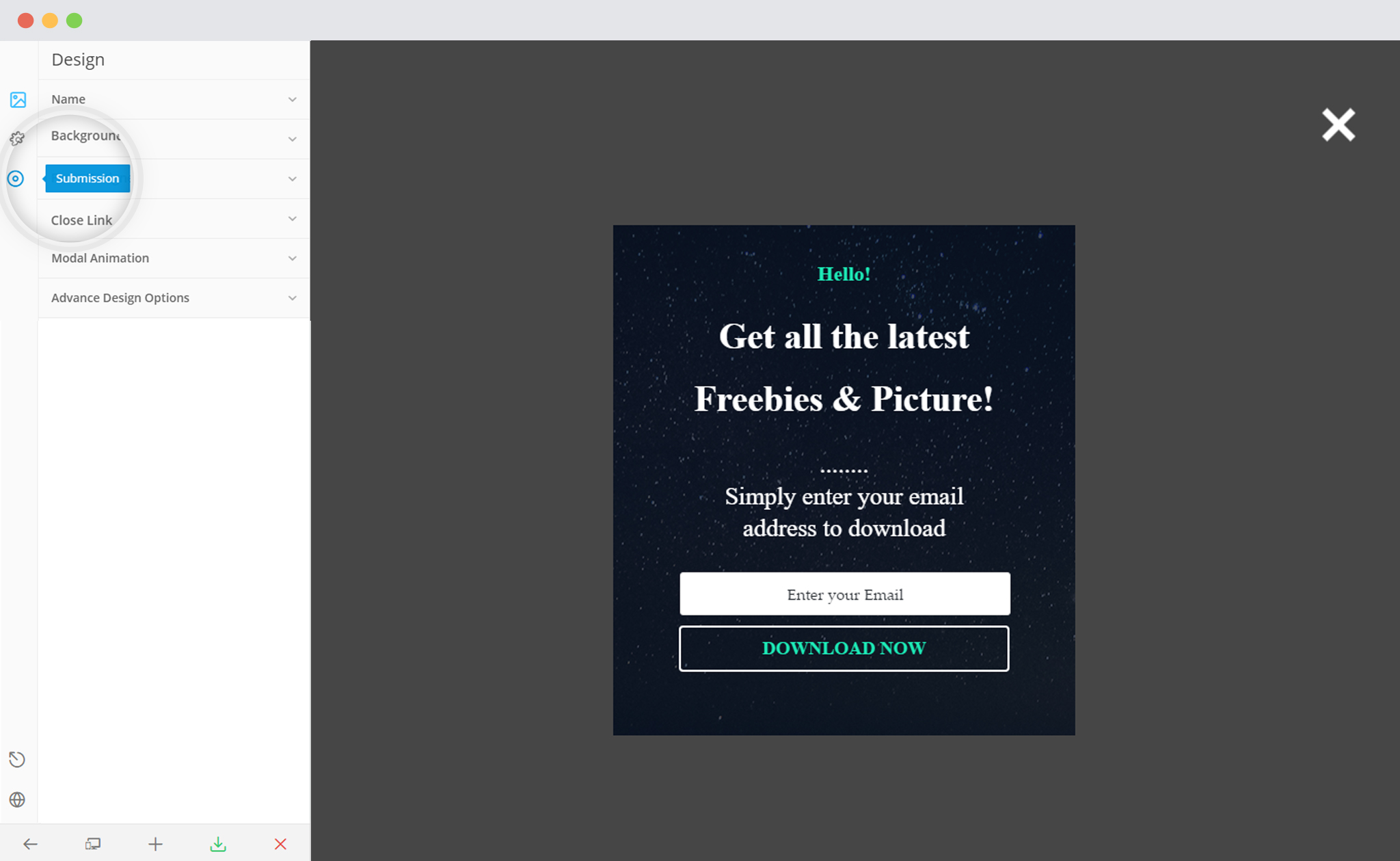The image features a series of intricately placed circles, including a red circle, a yellow circle, and a green circle, which together form a dynamic design. The background transitions from a gray shade to a smaller black segment, giving the design a layered effect.

At the center of this artistic composition, the word "Hello" is prominently displayed in green. Beneath it, there's a call to action encouraging viewers to stay updated with the latest freebies and images. This text is written in white and reads, "Get all the latest freebies and pictures, simply enter your email address to download." 

Below this instructional text is a white box where users are prompted to enter their email addresses, with the field label "Enter your email" displayed in black. The box is traced by a white outline, accompanied by a green "Download Now" button.

The top right corner of the image features a white "X," likely representing a close button. The entire layout suggests a modern, advanced design interface focused on user interaction and accessibility.